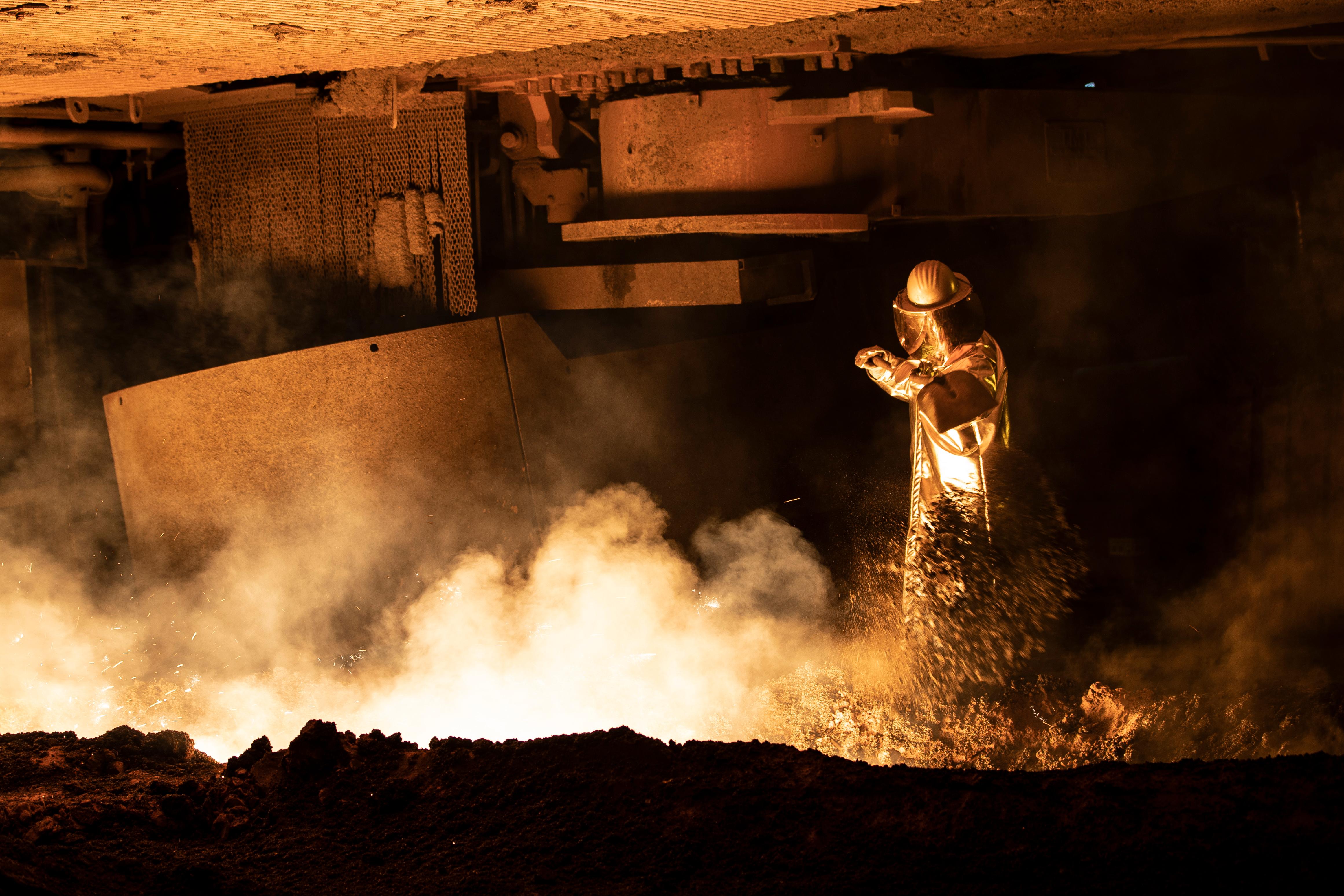In this image, we see a fireman, positioned to the right, fully equipped in his protective gear, including a helmet with a face shield and thick gloves, facing left. The setting appears to be inside a dark and somewhat eerie factory or warehouse, possibly underground. In front of the fireman, there is white smoke hovering near ground level, partially obscuring a bright, central fire with sparks flying, illuminating the surroundings. The bottom of the image features dark-colored dirt or clay, and some mud appears to be airborne near the fireman's waist. Behind the smoke, a metal board leans against a wall, and metal chains hang from the ripped-patterned ceiling. The backdrop contains various metal objects and tools, suggesting an industrial environment. The scene is devoid of text, with colors mainly consisting of muted tones such as black, brown, tan, white, yellow, and orange.